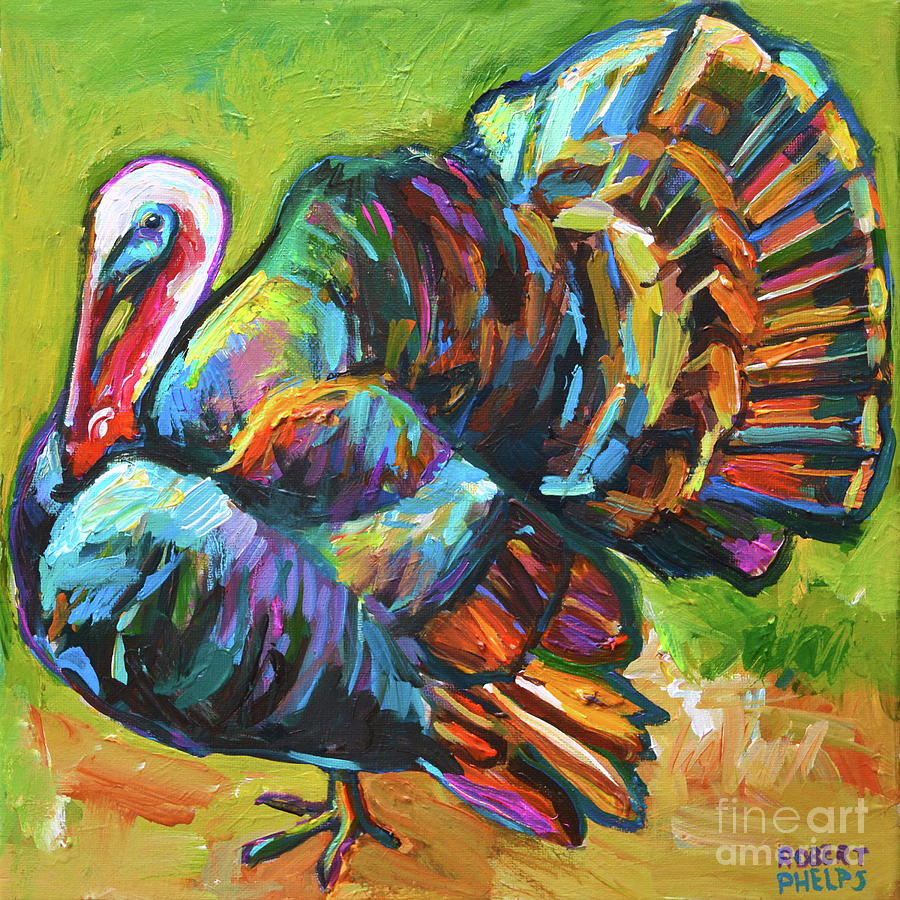This is an impressionistic square painting of a unique, multicolored turkey by artist Robert Phelps. The turkey, occupying almost the entire frame, is depicted with a dazzling array of colors. Its head is predominantly white with a pink outline and neck, complemented by a light blue face interspersed with purple, yellow, and green highlights. The large bird's black eye contrasts with its red beak. The turkey's body showcases a vibrant mix of blue, purple, orange, and green, blending into a predominantly brown rear. Both the tail and wings feature a striking pattern of adjacent rectangular strokes in a symphony of colors. 

The background, covering about three-quarters of the image, transitions from a smudged dark to light green with yellow highlights on the left, while the bottom portion transitions into earthy smudges of orange, yellow, and brown. The painting includes an artist's signature in the bottom right corner in purple all caps letters, "ROBERT," with "PHELPS" below it in blue. Just above the signature, there is a white watermark reading "FINE ART AMERICA."